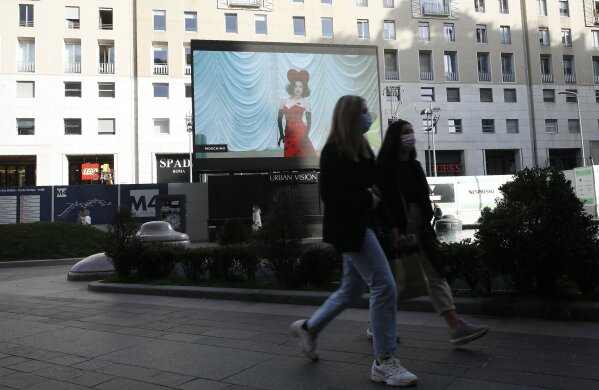The photograph, taken in a city during the daytime, showcases a bustling urban scene likely captured during the pandemic, as evidenced by two young girls in the foreground wearing surgical masks. These girls are walking along a stone walkway dotted with bushes and a median. The weather appears clear, as there are no umbrellas in sight.

Dominating the background is a large, multi-story building. The top half of the building is tan-colored and features windows with small balconies, likely indicating that it is an apartment complex. Below this, the building transitions to an off-white color, with large windows at ground level showcasing a couple of company advertisements.

Centrally positioned on the building is a large TV screen displaying an image of a woman of Caucasian descent. She is elegantly dressed in a red gown and matching headpiece, resembling Mickey Mouse ears, and is shown standing on a stage with a white, fancy drop-down curtain behind her. This screen grabs one’s attention amid the urban surroundings.